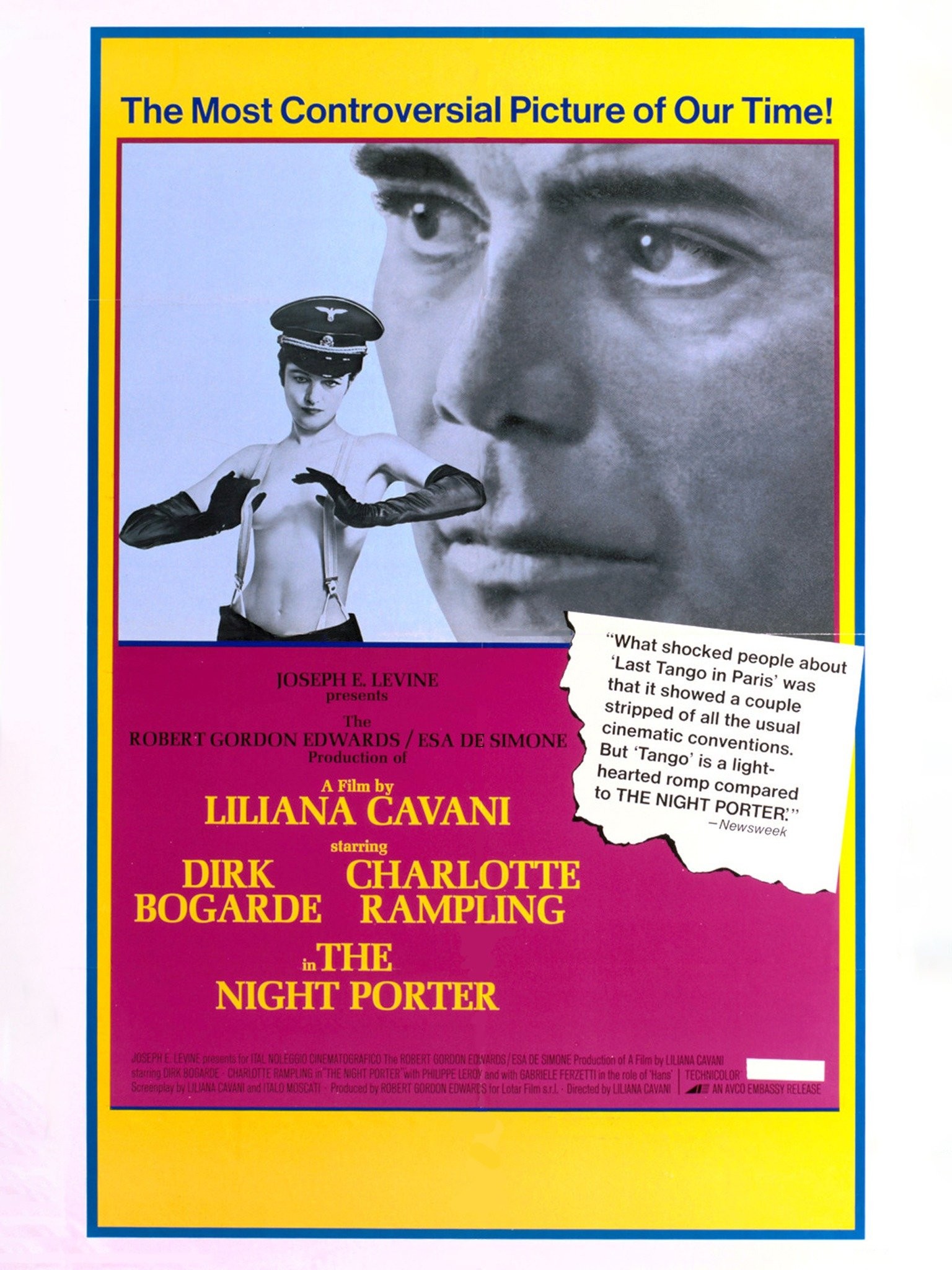The image is a detailed movie poster with a distinctive blue outline and a yellow body, featuring an inner section with a red border and a pink-magenta background. The title at the top declares, in blue text with an exclamation mark, "The Most Controversial Picture of Our Time." Below the title is a black-and-white photo of a woman wearing a German officer hat, long bicep-length gloves, and suspenders attached to her pants, using her fingers and hands to cover her bare breasts. Behind her, there is a close-up image of a man's face, with staring eyes, adding a mysterious element to the composition. The poster includes a quote from Newsweek Magazine, noting that "What shocked people about Last Tango in Paris was that it showed a couple stripped of all the usual cinematic conventions, but Tango is a light-hearted romp compared to The Night Porter." The film is presented by Joseph E. Levine, produced by the Robert Gordon Edwards/Isa De Simone production, and directed by Liliana Cavani. It stars Dirk Bogard and Charlotte Rampling, showcasing "The Night Porter" in bold, prominent text.